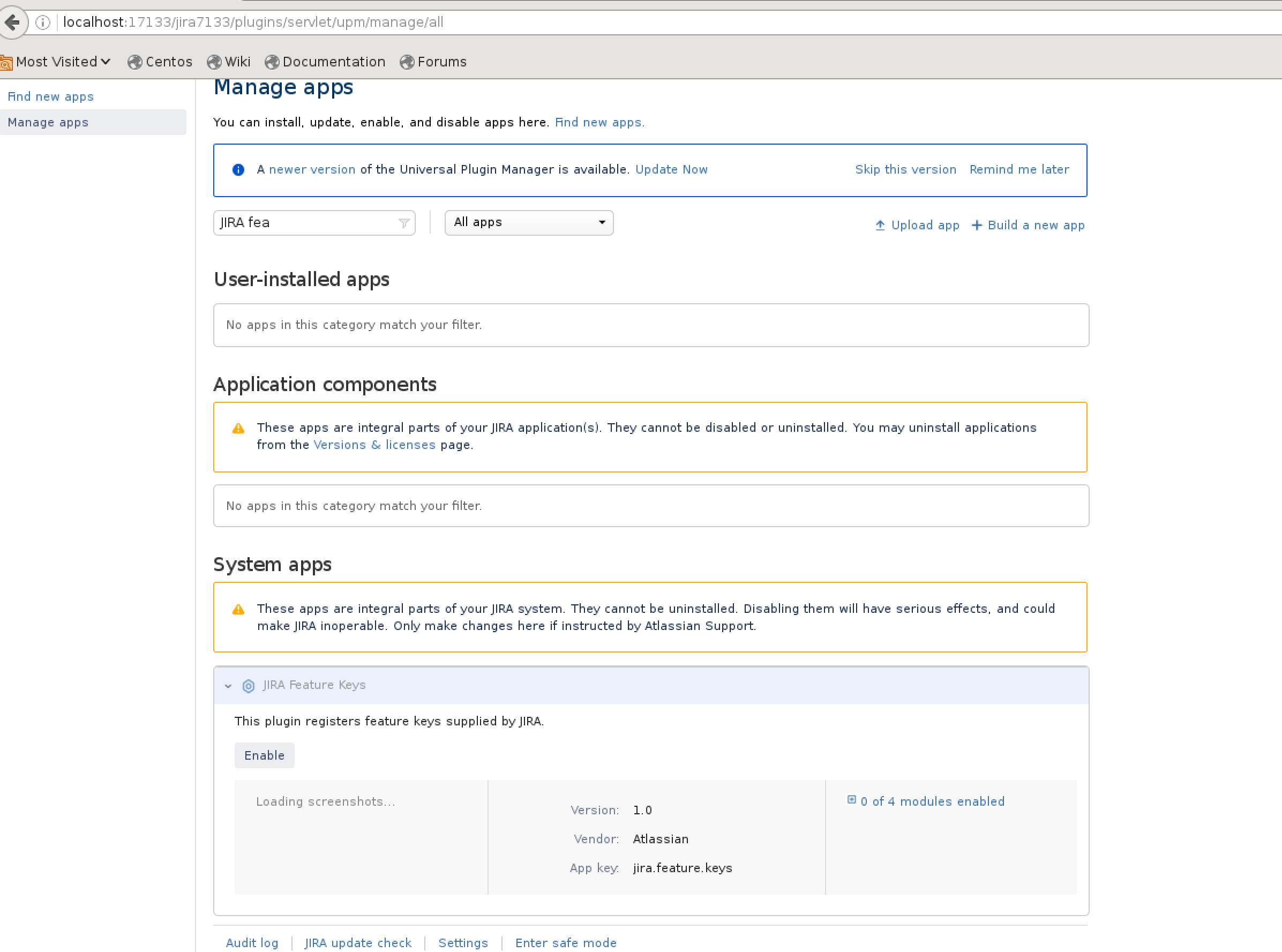This image depicts a web page titled "Local Host - Manage Apps." The page allows users to find, install, update, enable, and disable various applications. At the top, a prominently displayed blue link labeled "Find New Apps" invites users to discover additional apps. Below this, a blue box notifies users of a newer version of the Universal Plugin Manager, offering options to "Update Now," "Skip This Version," or "Remind Me Later."

Further down, there's a dropdown menu named "JRA fee," along with another dropdown labeled "All Apps." Users have the option to upload a new app or build one from scratch. A message indicates that there are currently no apps matching the selected filter within the "User Installed Apps" category.

The page also features a yellow warning box specifying that certain "Application Components" are essential to the JIRA applications and cannot be disabled or uninstalled. For further actions, users are directed to the "Versions and License Page" through a clickable blue link.

At the bottom, another message states that no apps in this category match the selected filter. Additionally, a blue box labeled "JRA Feature Keys" explains that this plugin registers feature keys supplied by JIRA, with an option to enable it. The page includes sections with gray boxes containing details about the vendor, version, and app key of each app, providing necessary technical information.

Overall, the page is designed for the comprehensive management of applications, ensuring users have clear and accessible options for app maintenance and updates.